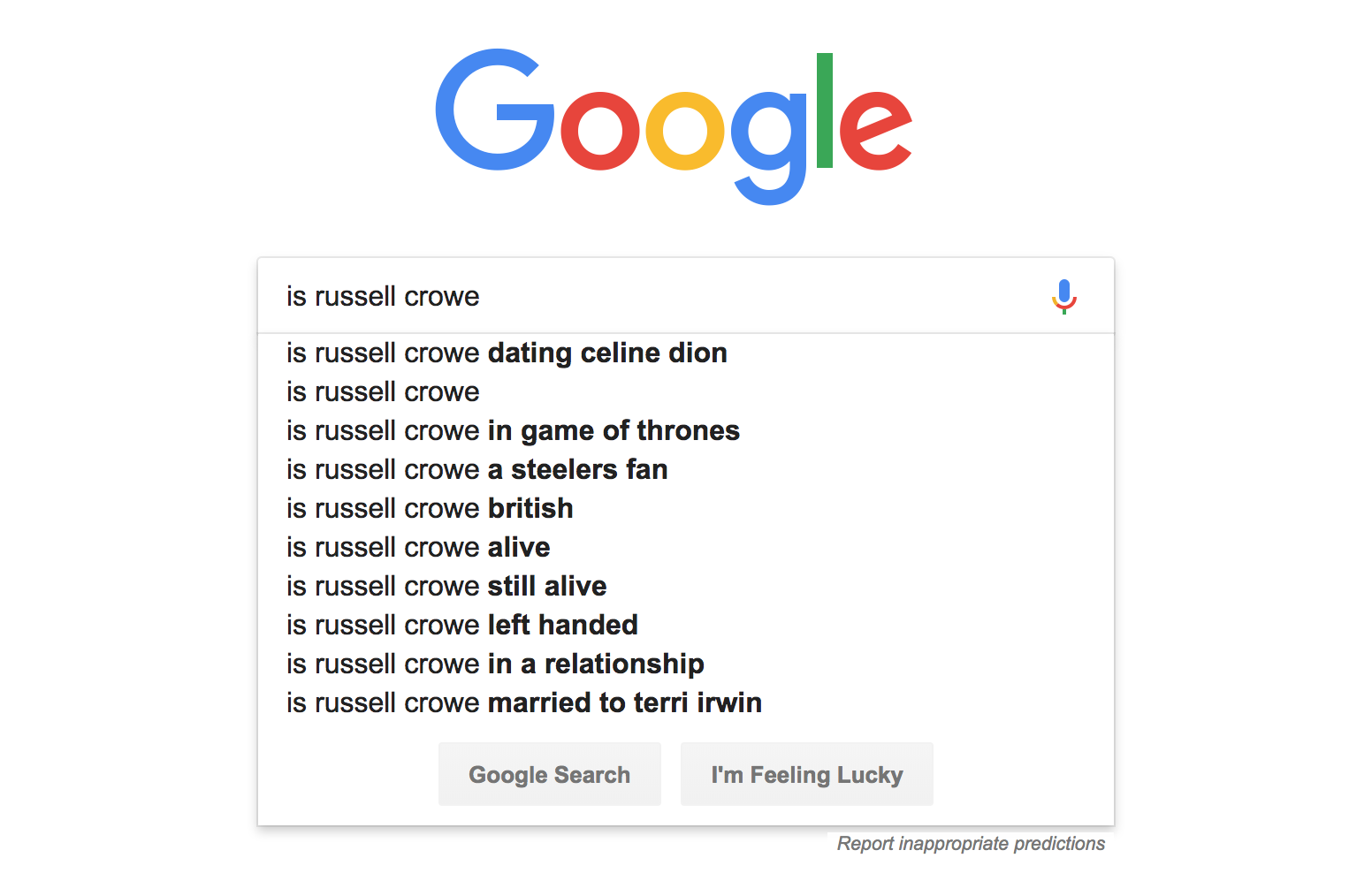A person is using Google search, and the displayed webpage focuses on the central area featuring the iconic Google logo and search bar. The Google logo at the top is spelled out with a blue "G," a red "O," a yellow "O," a blue "G," a green "L," and a red "E," all set against a white background. Beneath the logo is a horizontal search bar with a blue-and-red microphone icon on the right side. In the search bar, someone has typed "is Russell Crowe?" in bold black text. Below this, a drop-down list of related search suggestions is visible, helping refine the query. The suggestions include: "is Russell Crowe dating Celine Dion?", "is Russell Crowe?", "is Russell Crowe in Game of Thrones?", "is Russell Crowe a Steelers fan?", "is Russell Crowe British?", "is Russell Crowe alive?", "is Russell Crowe still alive?", "is Russell Crowe left-handed?", "is Russell Crowe in a relationship?", and "is Russell Crowe married to Terry Irwin?". Underneath the suggestions, there are two rectangular light gray buttons; the left button says "Google Search" in bold gray letters, and the right button says "I'm Feeling Lucky" in bold gray letters. Just outside the gray frame of the drop-down window, there is a light gray italicized text that reads "Report inappropriate predictions."